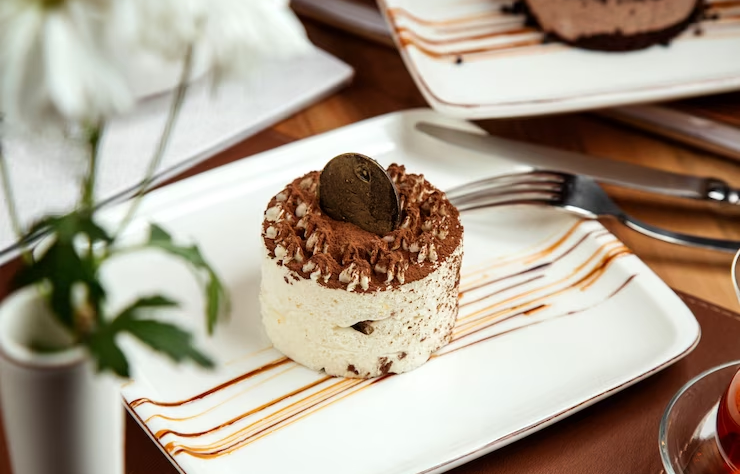A detailed image description of a dessert plate set in what seems to be a restaurant. In the center, a white square plate holds a round dessert that resembles tiramisu or a mousse, characterized by a light white base topped with chocolate shavings and cocoa powder. At the pinnacle of the dessert, a circular cookie or chocolate piece stands upright. The plate features drizzles of caramel and chocolate lines across its surface. A fork and a knife rest by the side of the plate. In the background, another similar plate with half a dessert is visible, though out of focus. To the side, a small white vase containing green foliage and white flowers is slightly blurred. The setting is atop a wooden table, possibly accentuated with a leather placemat. The colors in the image are primarily green, white, brown, tan, silver, and orange, with no textual elements or people present.